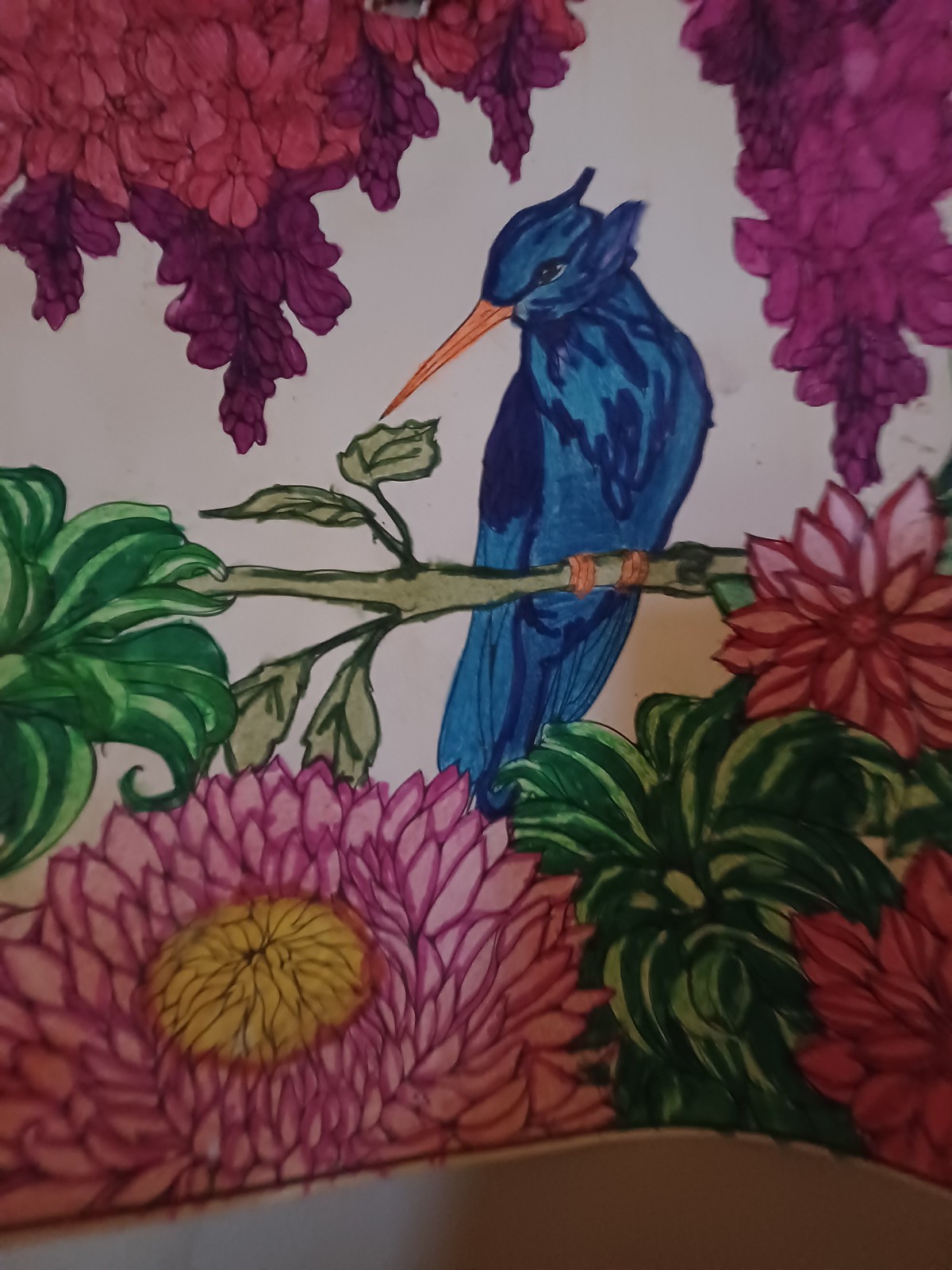This image, likely a photograph of a vibrant, marker-drawn artwork on white fabric or tapestry, showcases a blue hummingbird perched on a light green stem, reminiscent of a sunflower stalk. The bird, highlighted with a darker blue patch on its wing and small orange feet, faces the viewer but gazes leftward with its long, thin orange beak and distinctive feather "horns" above its head. Surrounding the hummingbird are a variety of colorful flowers: cascading clusters of pink and purple blooms at the top, magenta-shaded leaves and flowers in the corners, and notably, a zinnia at the bottom center featuring dark pink petals with lighter pink interiors and a yellow center, encircled by green foliage. This detailed and delicate scene is artistically rendered using colored markers.